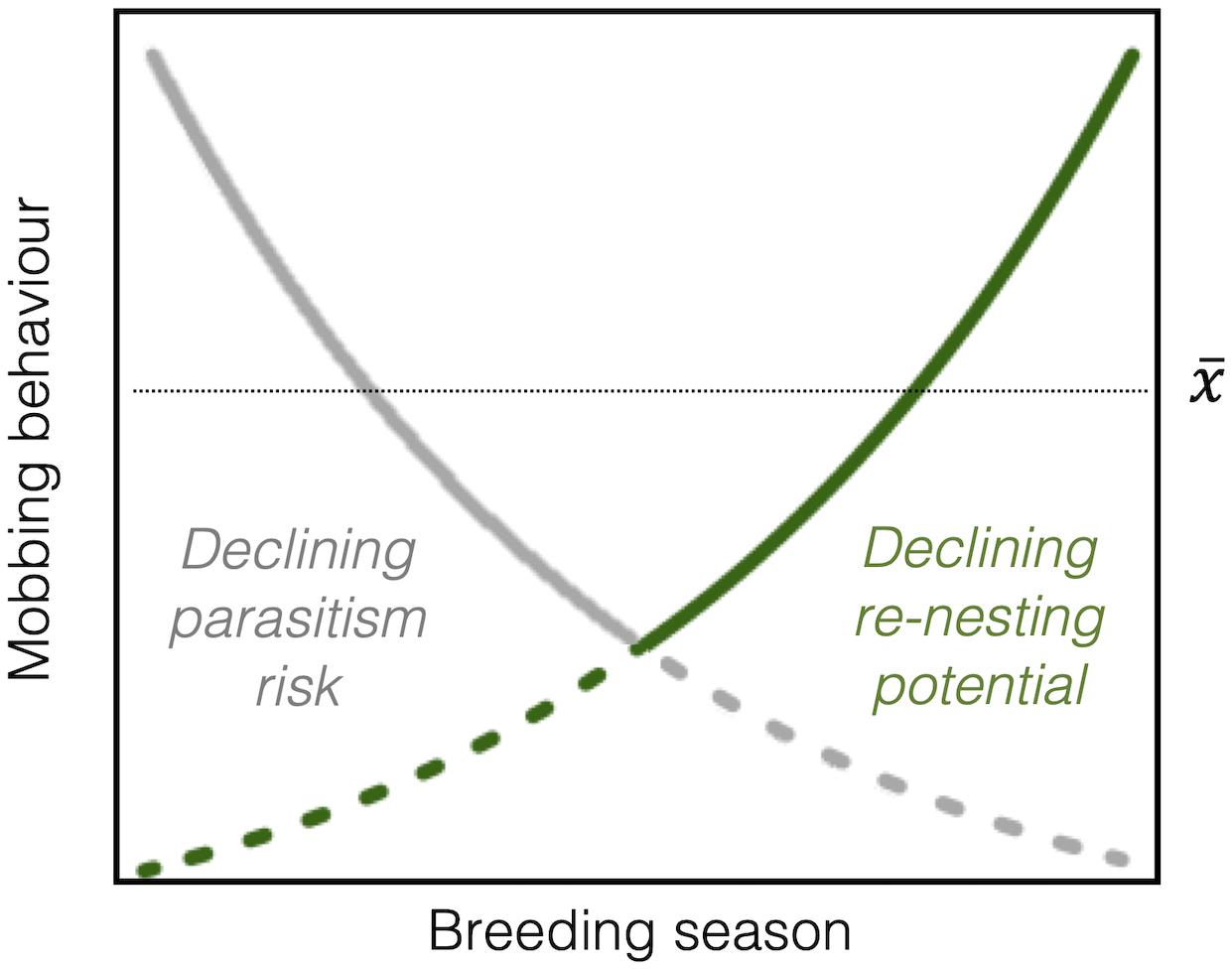The image is a detailed chart set within a black outlined square, representing a graph with distinctive axes. The vertical axis (y-axis) is labeled "Mobbing Behavior," and the horizontal axis (x-axis) reads "Breeding Season." Within the square, a gray line begins at the upper left corner, moving diagonally downward to the lower right. Halfway through its descent, the gray line transitions from solid to dotted. Mirroring this, a green line starts at the upper right corner, sloping diagonally downward to the lower left, and also switches from solid to dotted about halfway. A horizontal dotted line runs across the middle of the graph, dividing the area into two distinct zones. The lower part of the graph indicates “Declining Parasitism Risk” in gray text on one side and “Declining Re-nesting Potential” in green text on the other side.